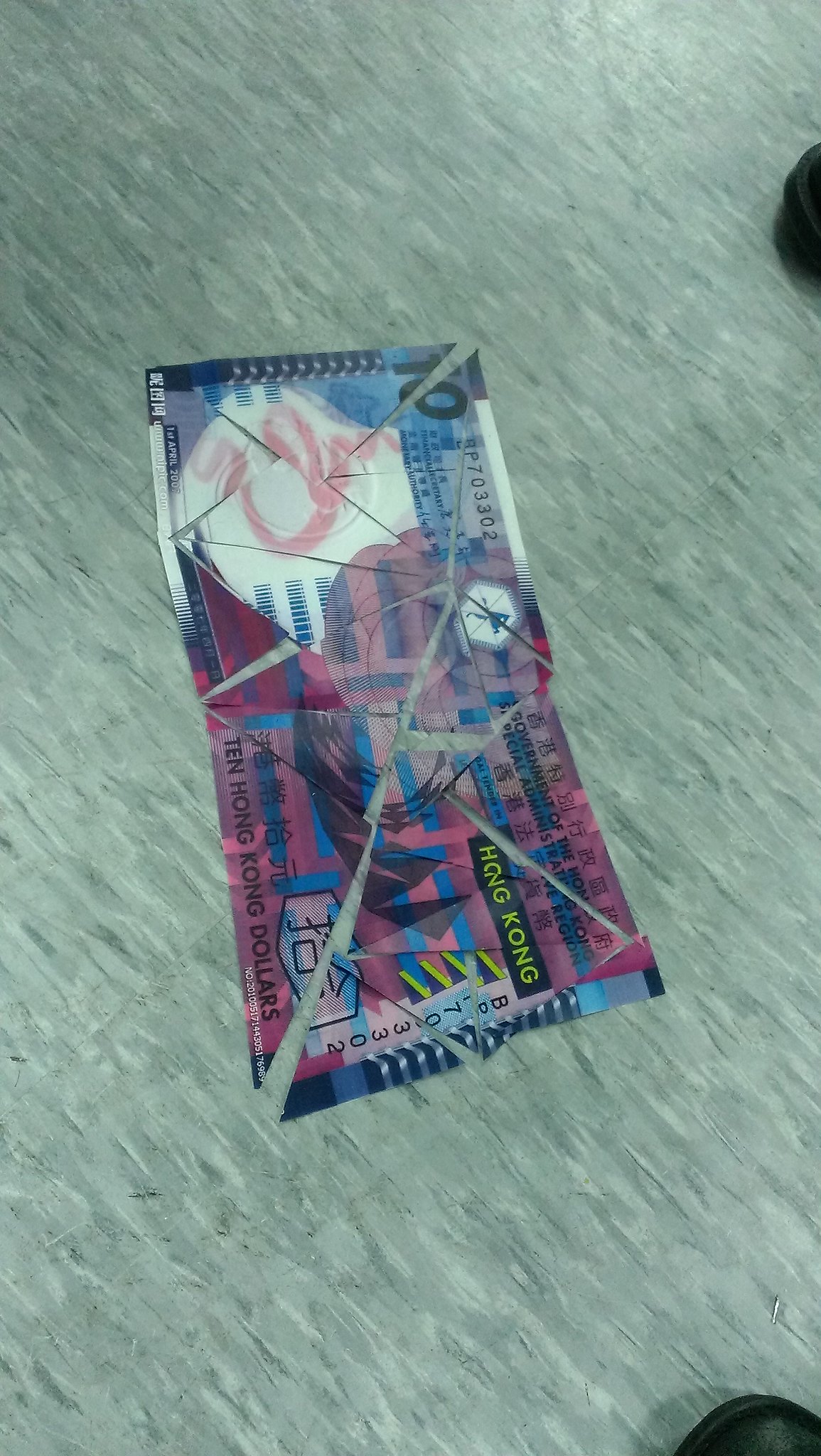At first glance, the image appears to be an intricately painted artwork, but upon closer inspection, it reveals itself to be a photograph. The photograph captures a tile floor with a green, gray, and beige pattern. On the floor lies a ten Hong Kong dollar note, meticulously cut into numerous triangles and then pieced back together, giving the appearance of a fragmented yet recomposed bill. At the edges of the photo, particularly the right edge and bottom right corner, we can see the tips of two different pairs of shoes with brown soles, belonging to different individuals. The composition and careful arrangement of the note's pieces, combined with the presence of the shoes, suggest a deliberate artistic intervention that transforms the mundane floor into a canvas of contemporary expression.